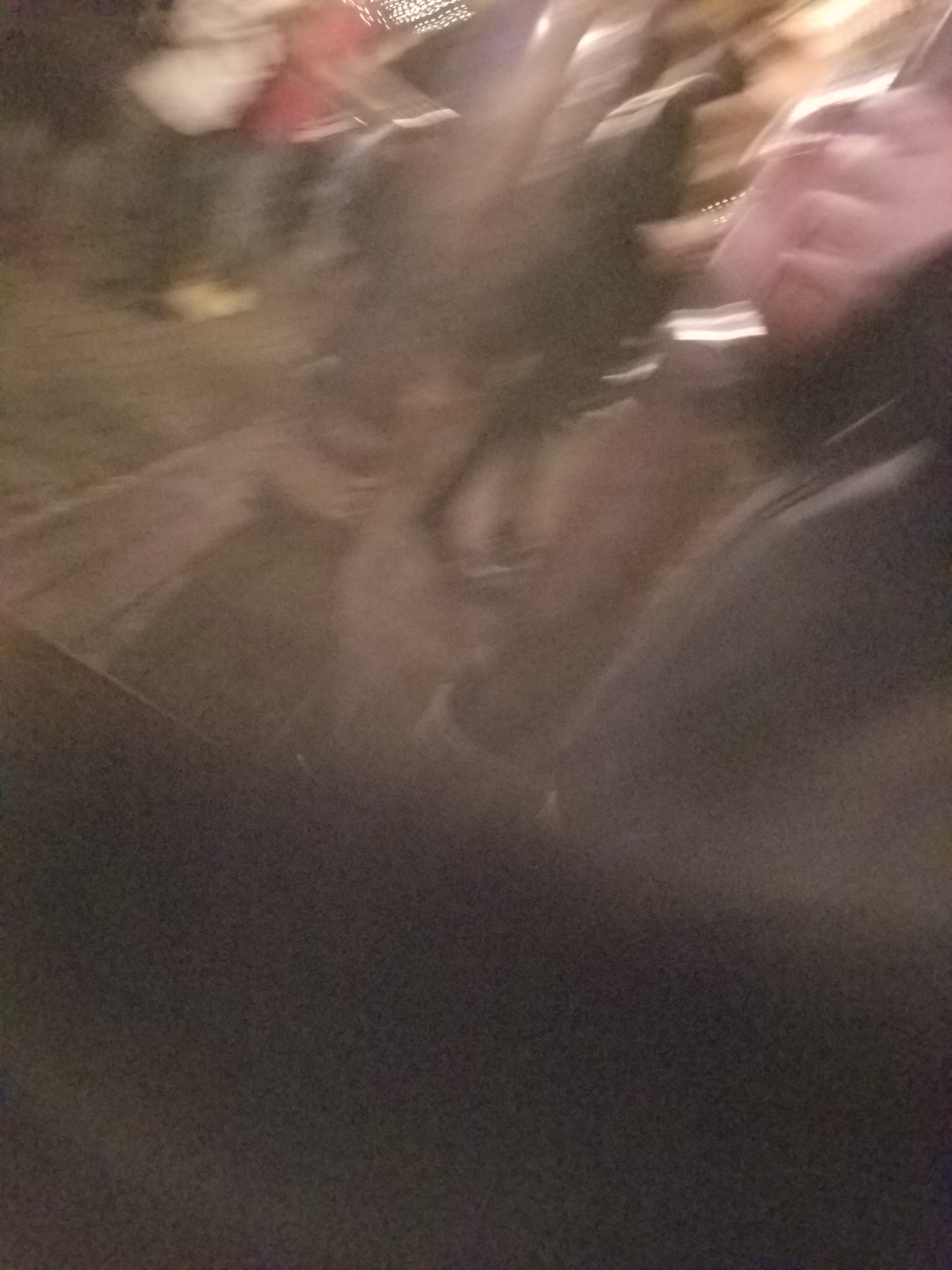This image appears to be a dark, heavily blurred photograph, potentially capturing a scene in rapid motion or compromised by poor quality. The lower part of the image is predominantly black, while the upper section features lighter shades. In the upper left corner, there seems to be a figure wearing a red shirt, jeans, and tan shoes, though it is difficult to discern due to the blurriness. Behind this figure, another individual in white is vaguely visible. To the right, a dark, indeterminate shape might represent another person or a shadow. Further right, a disproportionately large, blurry hand-like figure in a black sleeve stands out, adding to the overall confusion and surreal quality of the image.